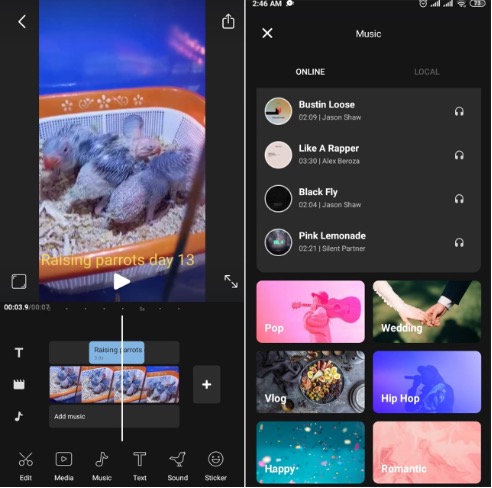The image is an intriguing split-screen display that appears to capture two mobile phone screenshots side by side. Both sides feature a black background.

**Left Screen:**
- The central focus is on four small, furry creatures that appear to be nestled in a little tray, potentially within a tank, as indicated by the glass reflection. A bright light shines overhead, possibly a heat lamp. The text "Raising parrots day 13" is prominently displayed.
- There are various UI icons: at the top, a left arrow (back button) and a send icon (depicted by a piece of paper with an arrow). At the bottom left, a blank square, and at the bottom right, two arrows pointing northwest and southeast.
- Below this, a section that resembles video editing software shows the text "Raising parrots" in blue, along with a timeline that indicates the video is three seconds in. Several icons are visible including a 'T' (text), calendar, and a music note, plus the option to "add music" and a '+' sign.
- Menu options at the very bottom include: "edit" (scissors icon), "media" (play button), "music" (music note), "text" (T), "sound" (bird), and "sticker" (smiley face).

**Right Screen:**
- At the top, indicators show it's 2:46 a.m., the alarm is set, the broadband signal is strong, and the battery is either at 23% or 73%.
- A white X and the word "Music" lead into a playlist featuring songs such as "Bustin Loose" by Jason Shaw, "330" by Alex Baroza, "Black Fly" by Jason Shaw, and "Pink Lemonade" by Silent Partner. Each song is accompanied by album art and a pair of headphones icon.
- Below the playlist, there are different music categories: "pop" (image of someone with a guitar), "wedding" (groom and bride holding hands), "vlog" (food on a table), "hip-hop" (hip-hop artist), "happy" (confetti falling into a pool), and "romantic" (pink and swirly background).

Overall, this detailed and multi-faceted image offers a comprehensive look into both a video in progress about raising parrots and a curated music selection for video editing.